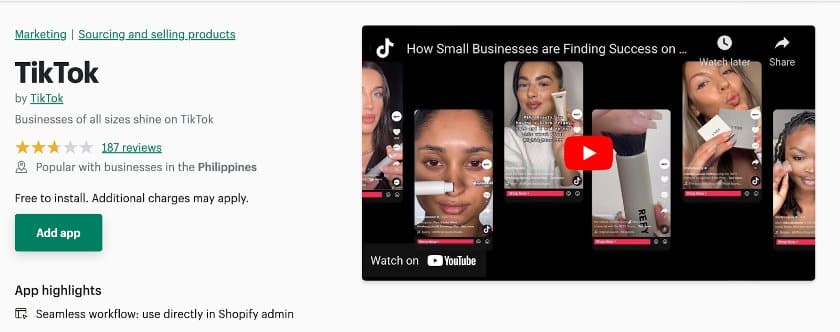**Caption:**

The image is a detailed interface on integrating TikTok with Shopify for businesses. 

**Left-Hand Side:**
- **Top Left:** The TikTok logo with the heading "Marketing and Sourcing and Selling Products" in blue, coupled with TikTok's signature color.
- **Subheading:** "Business of all sizes shine on TikTok" in gray.
- **Ratings and Reviews:** Displayed as three stars out of five, based on 187 reviews.
- **Target Audience:** Noted to be popular with businesses in the Philippines.
- **Cost Indication:** Stated as "Free to install," though additional charges may apply.
- **Call to Action:** Presented in a green square button that says "Add App."

**Highlights Section:**
- Emphasizes a "Seamless workflow used directly in Shopify admin."

**Right-Hand Side:**
- **YouTube Video Interface:**
    - The TikTok logo is located at the top left.
    - A red square with the play icon is centered within the video thumbnail.
    - Title: "How small businesses are finding success on..." followed by an ellipsis.
    - Thumbnails: Features six individual phone screen images of different women using makeup products.
    - Top right icons: Include "Watch Later" and "Share," both in white.
    - Bottom left: A "Watch on YouTube" prompt on a black background.

This comprehensive layout visually represents how businesses can utilize TikTok for marketing within the Shopify admin, accompanied by a video showcasing the success stories of small businesses.